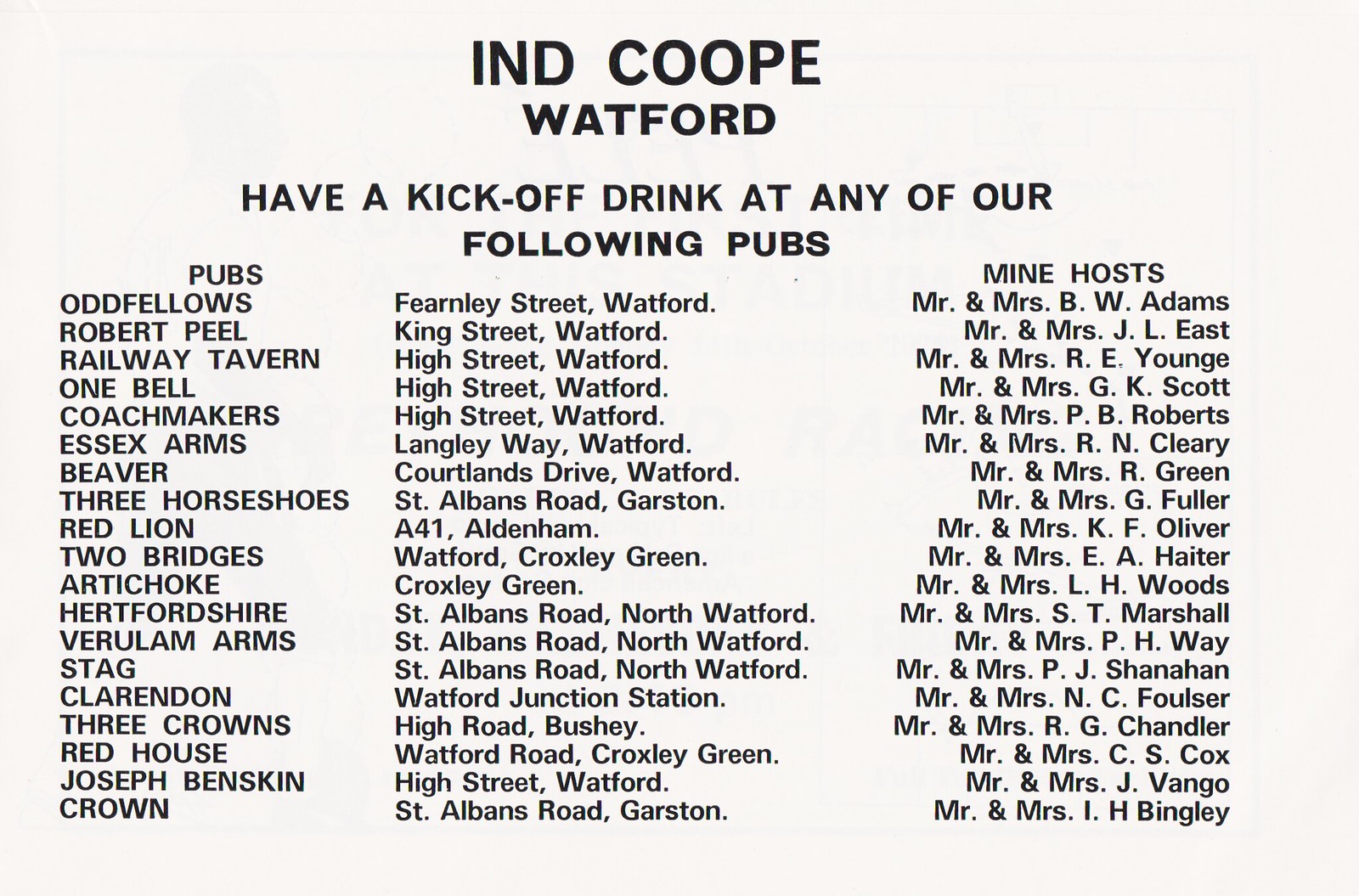The image is an informational sheet featuring a black and white design, with the title "IND Coop, Watford" centered at the top in all caps. Below the title, the text reads "Have a kickoff drink at any of our following pubs." The sheet is organized into three columns: the left column lists the pubs, the center column provides the locations, and the right column, titled "Mine Hosts," lists the hosts for each pub, all starting with "Mr. and Mrs." There are approximately 15 to 20 pubs listed, including Oddfellows, Robert Peel, Railway Tavern, One Bell, Coachmakers, Essex Arms, Beaver, Three Horseshoes, Red Lion, Two Bridges, Artichoke, Hertfordshire, Furloom Arms, Stag, Clarendon, Three Crowns, Red House, Joseph Benskin, and Crown. Specific details include that Crown is located on St. Albans Road, Garston, with hosts Mr. and Mrs. I.H. Bingley, and that Two Bridges, located in Watford, Croxley Green, is hosted by Mr. and Mrs. E.A. Hayter.